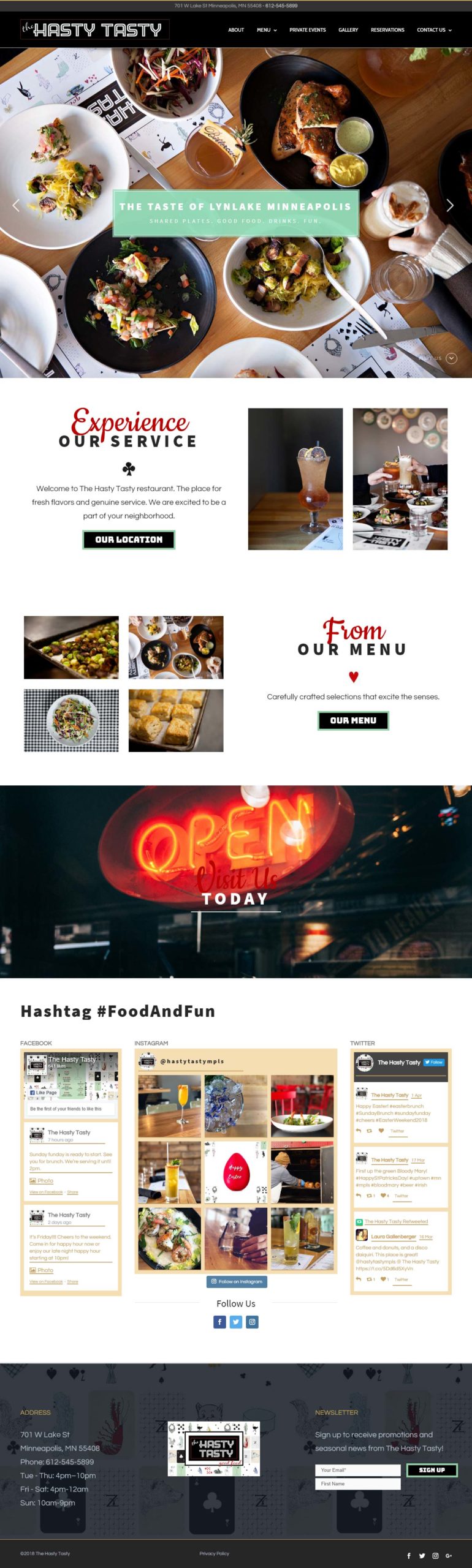The webpage displayed is a full-screen capture of the homepage for Hasty Tasty, a restaurant branding itself with the tagline "The Taste of Lynn Lake, Minneapolis." The central background is a high-resolution, top-down photograph of a table adorned with an array of dishes, giving potential diners a teaser of their diverse menu.

At the forefront, a mint-colored box featuring off-white text introduces the site. The navigation of the page employs a predominantly white background with black and red accent colors, enhancing a cozy and inviting aesthetic.

Headings such as "Experience Our Service" and "From Our Menu" are prominently showcased, accompanied by interactive buttons for locating the restaurant and exploring the menu. Though smaller text is present under these headings, the fine print is difficult to discern.

Scattered across the page are various images, including drinks, shakes, and meal options, which cleverly showcase the restaurant's offerings. Below the primary sections, a bold header stating "Open Today" catches the viewer's attention, followed by the unique hashtag "#foodandfun," encapsulated in text.

The website also integrates social media elements, likely linked to Instagram and Twitter, providing a glimpse into their online presence and community engagement. The footer consolidates essential links and information, and offers a newsletter signup option on the bottom right corner, inviting visitors to stay updated with Hasty Tasty's latest news and promotions.